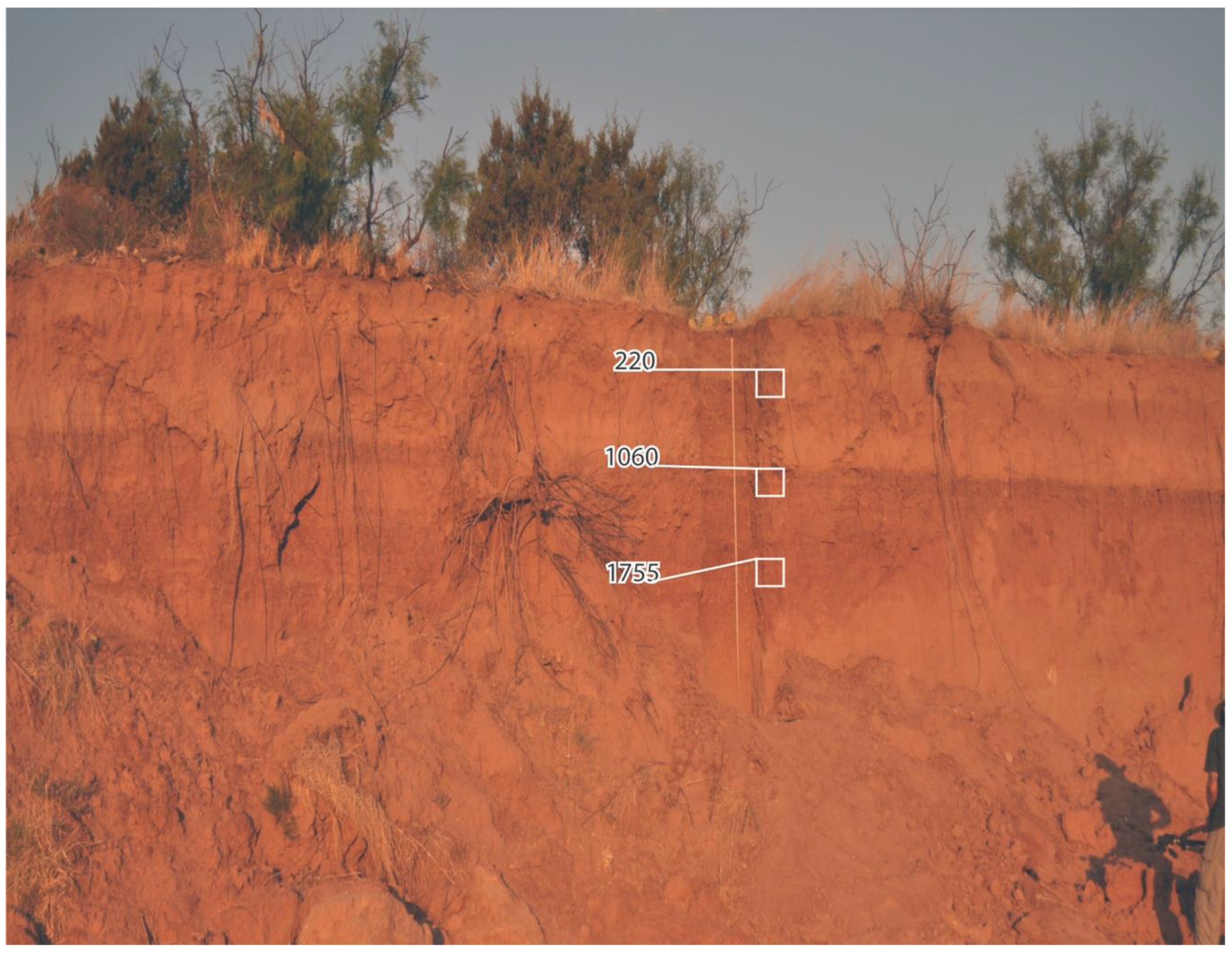This photograph captures a detailed cross-section of a reddish-brown cliff, potentially resembling the sedimentary layers found in areas like Arizona. The cliff, appearing to be 10-20 feet tall, is sharply cut, revealing various layers of soil, some light and others darker red. Green bushes and a few evergreen trees with a backdrop of a light gray, blue-gray sky crown the top of the cliff. Superimposed onto the image are digitally added annotations that identify distinct layers of sediment. At the top is a label marked "220," followed further down by "1060," and then "1755," each accompanied by white boxes and lines that designate specific soil layers. These markings likely indicate the relative age of the soil discovered at each depth. Near the bottom right corner, the shadowy figure of a man in beige pants and a black short-sleeved shirt is partially visible, standing on the edge of the image and casting a shadow on the red dirt. The overall scene presents a realistic, detailed snapshot of geological strata, possibly aimed at illustrating changes in soil composition over time.